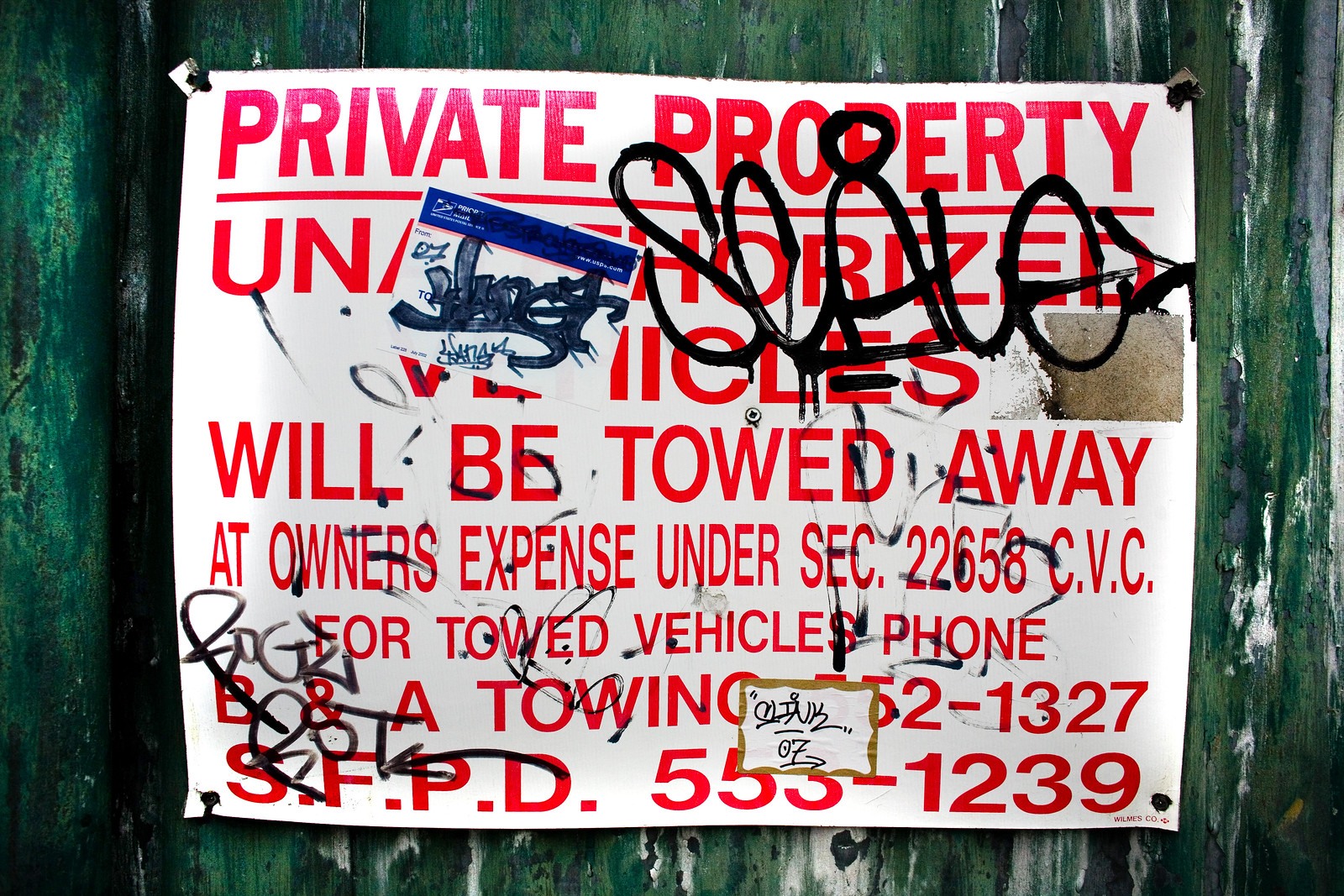The image depicts an old, worn wooden fence, featuring a heavily vandalized "Private Property" sign that is affixed to it. The fence exhibits a rough, aged appearance with chipped paint in shades of gray, green, and blue. The sign itself has a white background and bold red letters and reads: "Private Property. Unauthorized vehicles will be towed away at owner's expense under SEC 22658 CVC. For towed vehicles, phone B&A Towing at 352-1327. SFPD 553-1239." The sign is heavily defaced with black graffiti, including the word "SCALE" scrawled across the top right corner. There is also a "Hello, my name is" sticker with unreadable text in a fancy script, and various other errant black marks. A mail stamp is affixed across the word "unauthorized," adding to the sign's weathered and beaten appearance.